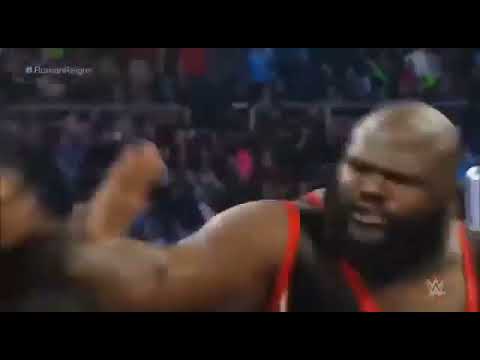The image depicts a high-energy moment captured in a blurry screenshot from a video, likely during a wrestling or boxing match set in an arena. Positioned near the right side of the frame is a muscular African-American man with a bald head and a prominent dark beard. He is wearing a sleeveless black shirt or tank top accented with red trim. His intense, fierce expression suggests he is either in the process of hitting someone or is about to strike. His arm, appearing blurred due to motion, is outstretched towards the left side of the image. The background, which is out of focus, features what seems to be a large crowd seated on bleachers, adding to the atmosphere of a live sports event. Additionally, a barely visible letter "W" can be seen in the lower right corner, hinting at the possibility that the image is a broadcast screenshot. The top and bottom of the image have horizontal black strips, framing the action-packed scene.